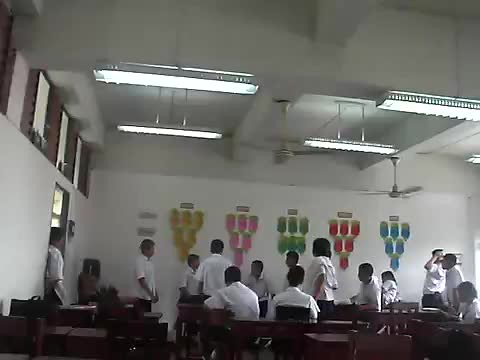The image depicts a predominantly white room with a minimalistic design. Along the back wall, five B-shaped objects are prominently displayed, each in a different color: yellow, pink, green, red, and blue, arranged from left to right. The space is occupied by several individuals, all wearing white shirts and sporting dark hair. These people are seated on wooden chairs equipped with round desks in front of them, while a few others are standing next to the colorful B-shaped objects. Ceiling-mounted are four visible long rectangular lights, with a fifth partially visible in the upper right corner. On the left side of the room, windows are positioned above a doorway, near which one person is standing. The overall ambiance of the room is bright and orderly, with a clear focus on the colored B-shaped items and the people interacting within the space.